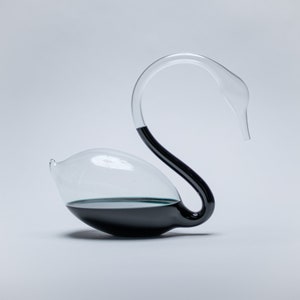The photograph captures a well-illuminated, clear glass object resembling a swan, set against a white background. This swan-shaped object appears to be a decanter, possibly used for wine. The swan's head curves gently downward, positioned to the right in a profile view. Within the swan's bulbous body and extending halfway up its neck, there is a very dark, almost black liquid, filling approximately 25% of the decanter. The rest of the neck and head remain empty. The detailed lighting provides a distinct shadow beneath the swan, enhancing its elegant, reflective surface.